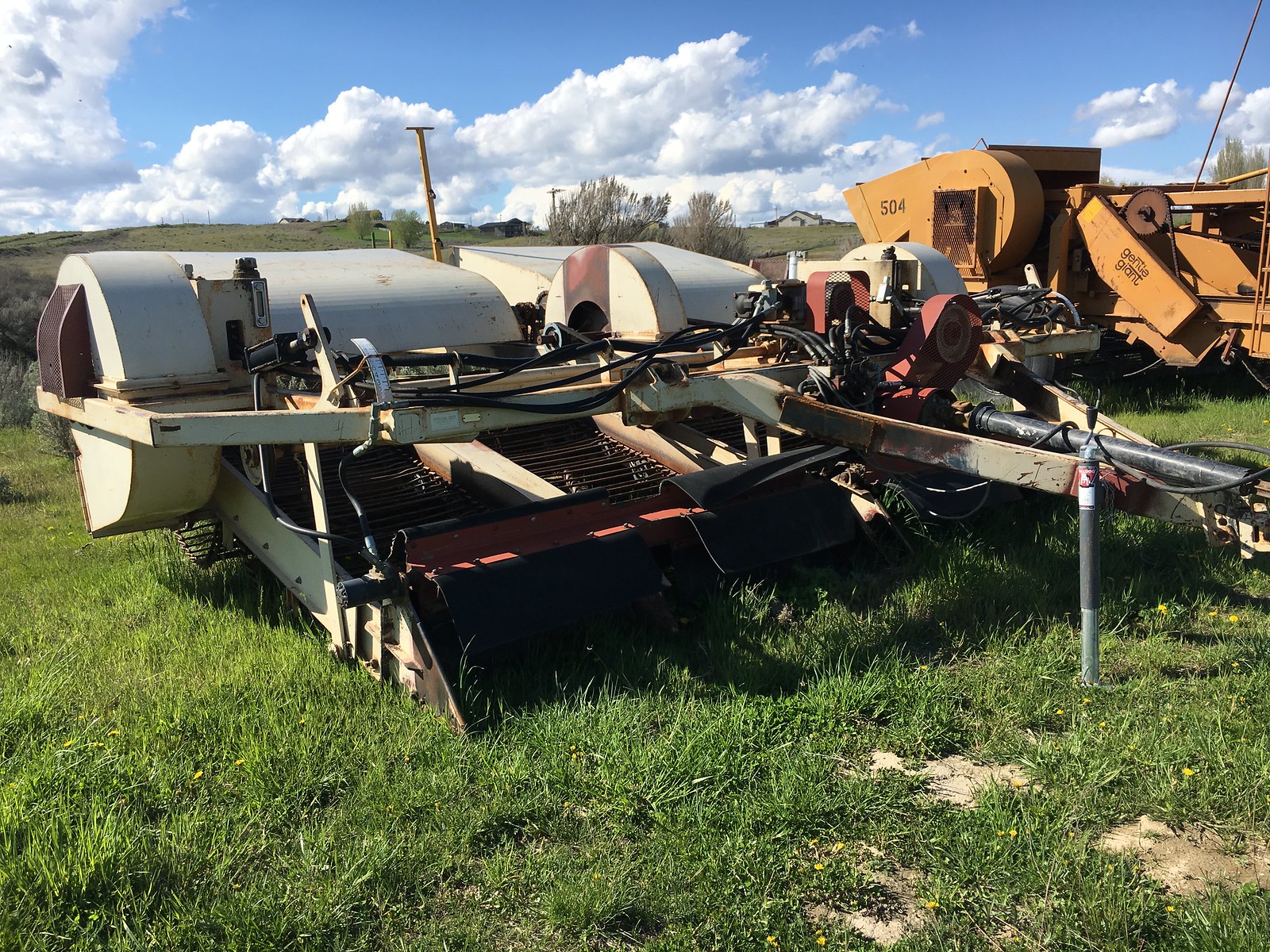The image depicts various pieces of farming equipment positioned on an expansive, grassy field. The scene features a mix of thick patches of grass interspersed with areas of exposed dirt. Two white machines with roller-like attachments, designed for scooping and scraping the ground, stand prominently in the foreground. Beside them, a distinctive yellow machine, branded as "Gentle Giant" with the number 504 visible, appears capable of picking up and possibly mulching materials. This machinery is likely used for agricultural or construction purposes. The setting is rural, with a vast expanse of green fields and some distant houses suggesting a residential development in the far background. A gentle hill can be seen rising towards the back of the image, framing a blue sky dotted with cumulus clouds, indicating a clear and pleasant afternoon.